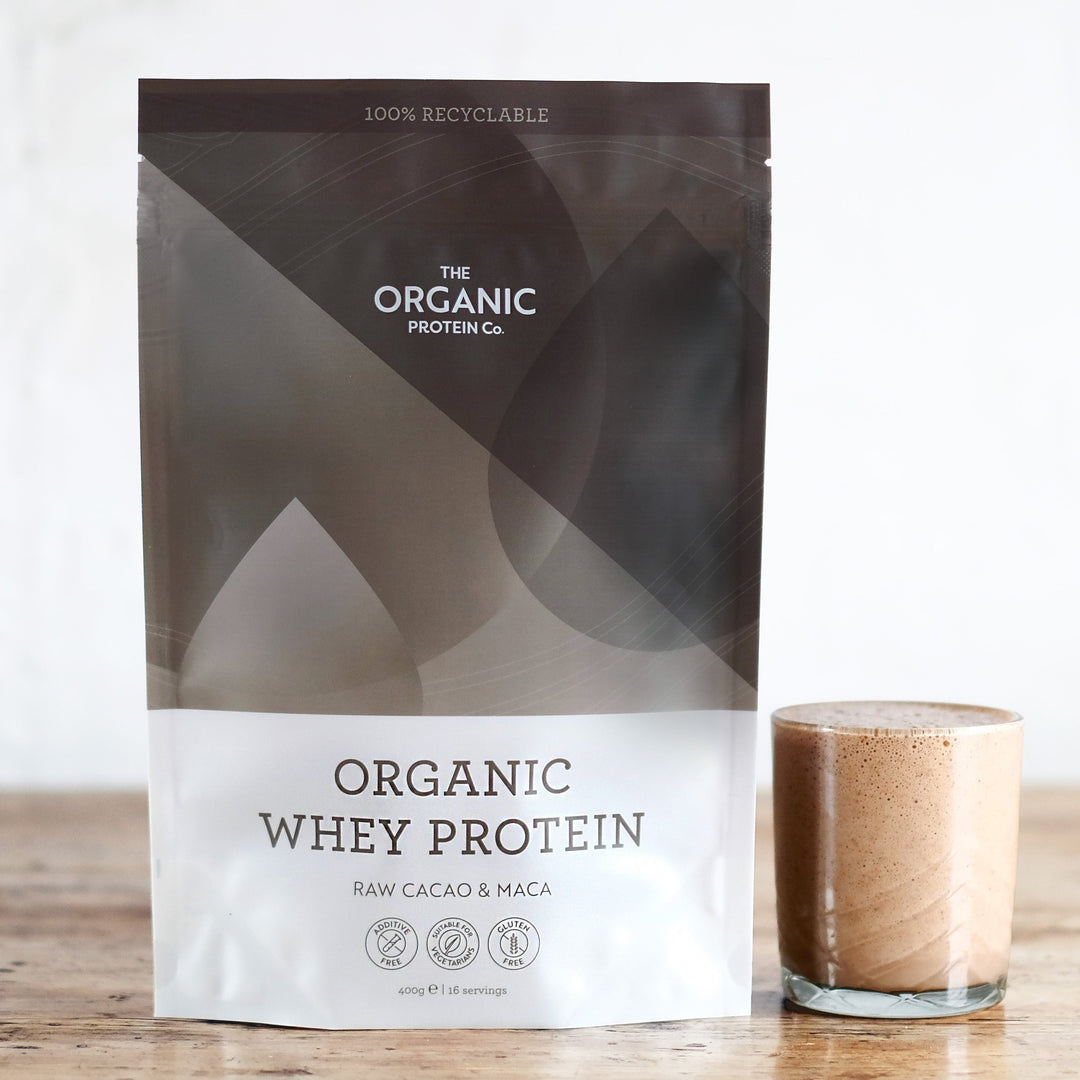This advertisement image features a bag of organic whey protein placed on a light-stained wooden table against a white background. The bag's design includes a distinctive gradient gray section at the top, divided diagonally from the top right to the lower left, creating a dark gray triangle on the left and a lighter gray triangle on the right. Above the indent tabs for the pull strip, there's a "100% recyclable" label in white on the dark gray triangle. Overlapping circles in varying shades of gray add subtle texture to the bag's design.

In white text on the lighter gray portion, "The Organic" is prominently displayed, leading down to an even lighter gray teardrop. At the bottom, the bag transitions to white, where "Organic Whey Protein" is printed, followed by the flavors "Raw Cacao and Matcha." Below this, three circular symbols indicate that the product is additive-free, suitable for vegetarians, and gluten-free. Additional text at the bottom reads "400 grams" and "16 servings."

To the left of the protein bag, a clear cup filled with a foamy, tan-colored shake—presumably made from the whey protein—is visible. The clear glass is shorter than the bag, providing a complementary visual element that emphasizes the product's use.